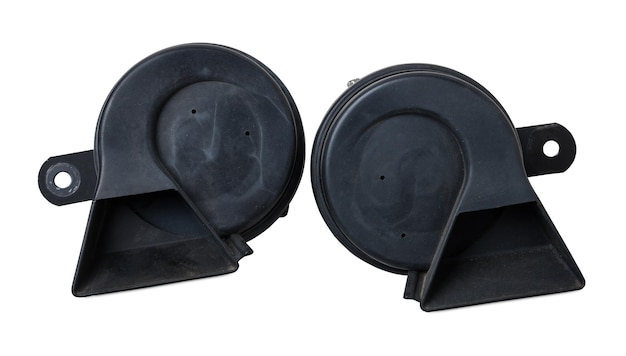This image showcases two nearly identical dark gray to black plastic devices, set against a plain white background. Each device has a circular main body that transitions into a trapezoidal shape at the bottom, where the black plastic flares outward, creating a darkened patch. Both items have noticeable signs of wear, giving them a brushed, roughed-up appearance. The devices appear to be mirrored versions of each other, with one facing left and the other facing right. They both feature a small half-oval extension on the sides, each containing a circular hole, possibly for mounting purposes. Resembling components like horn buttons for steering wheels or wheel covers for chair legs, these items suggest functionality and potential industrial application.